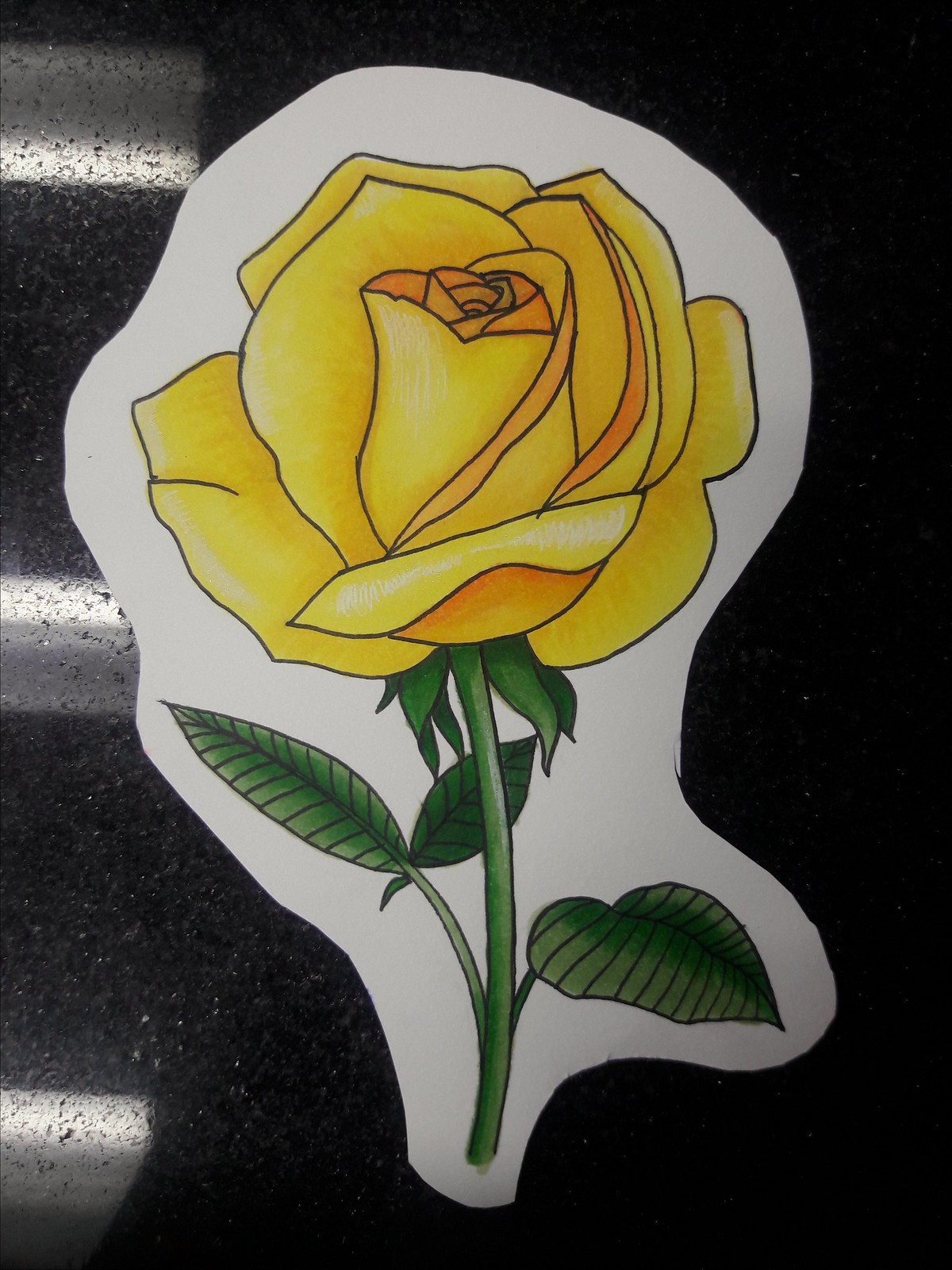This is a meticulously hand-drawn illustration of a vibrant yellow flower with a green stem. The flower, complete with delicately rendered petals, sits on a piece of white paper that has been expertly cut to match the flower's footprint. The drawing is distinguished by its intricate details, including fine black veining on the green leaves and a precise black outline around both the petals and the stem. The white paper, with its beautifully crafted floral design, rests on a dark, speckled surface that features reflective white spots, adding a subtle contrast to the composition. The overall effect is a striking and elegant presentation of the flower, highlighted by the careful attention to detail in both the drawing and its display.